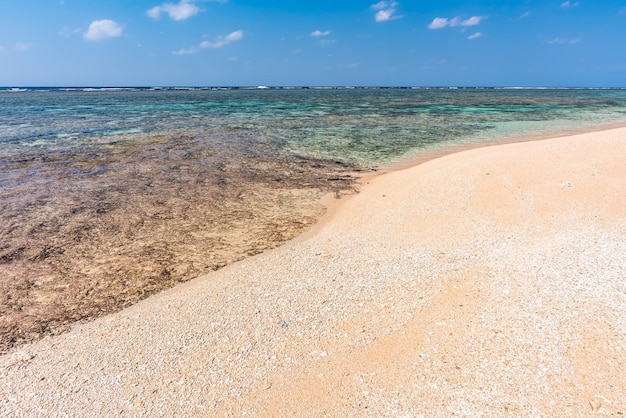This image captures a sandy beach with a distinctive pinkish hue, transitioning into fine light brown and coarse white sand scattered with small white rocks. The sand forms a diagonal line starting from the bottom right, stretching upward toward the center, and continuing to near the top right. As the beach meets the water, the shore appears dirty with dark brown foam and seaweed, creating a stark contrast against the otherwise tranquil setting. The water, in hues of light to dark turquoise green, laps gently against the sand without forming wave caps. However, farther out at the coral reef's edge, continuous waves stretch across the horizon. Overhead, a partly cloudy blue sky completes the serene yet slightly blemished seascape.